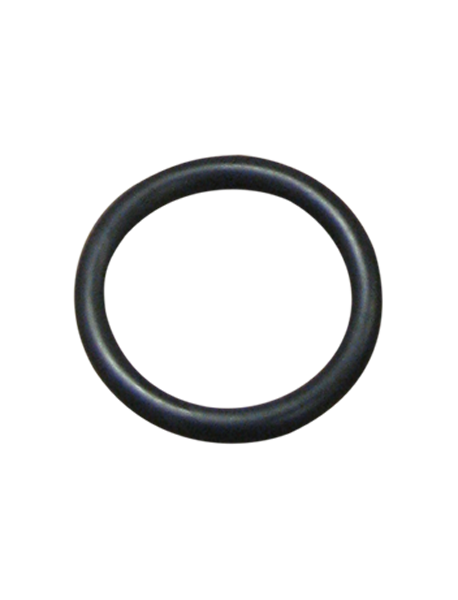The image features a very simple, yet detailed product photo of a black rubber O-ring, likely meant for plumbing. Central on a pristine white background, this completely circular rubber seal is depicted with precision. The top of the ring reflects overhead light, creating a grayish sheen that contrasts with the entirely black, matte-finished surface. While its exact size is indeterminate due to the lack of scale references, the lighting accentuates the rounded shape, casting subtle shadows within the interior circle. This professional product image, reminiscent of those seen in online marketplaces like Amazon, showcases the O-ring's potential utility in repair or assembly tasks.